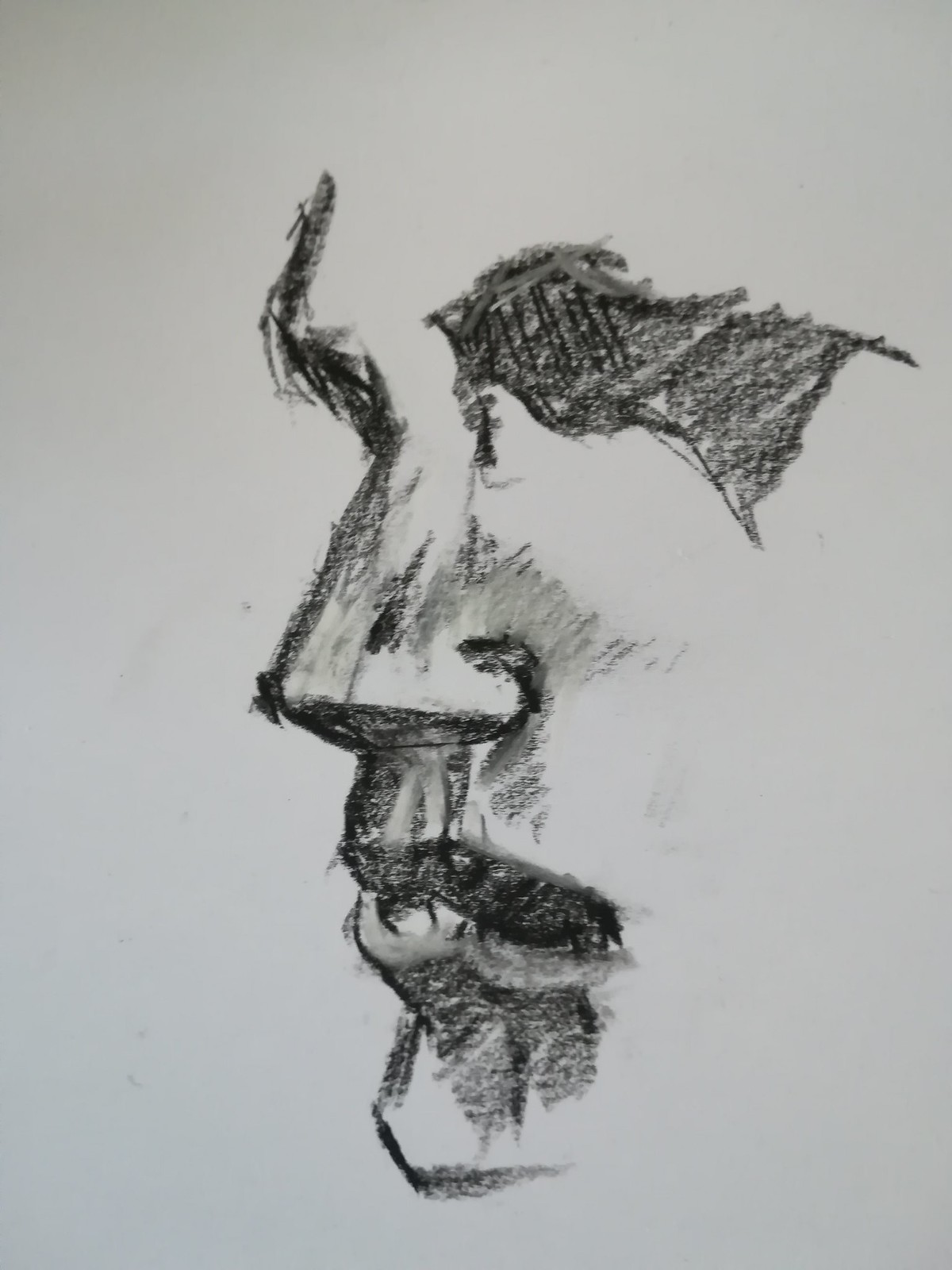This image is a crayon drawing characterized predominantly by the use of a black crayon, which adds an intense contrast to the composition. At the center of the artwork, there appears to be a chalice or a torch, which is ambiguously depicted. It is gripped by a hand that exudes a sense of strength and determination. Surrounding the central figure is a mysterious horse-like form, its presence adding an air of mystique and mythological intrigue. The lines are bold and deliberate, showcasing the artist's expressive use of the medium. The interpretation of the image may vary, invoking elements of fantasy and symbolism.